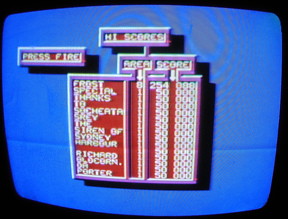A black-rimmed TV screen prominently displays a blue background, showcasing a high-score leaderboard from a video game. The list of high scores is clearly visible, with names and corresponding scores neatly arranged. At the top of the list is "Frost," with an impressive area score of 254,000, formatted as "254 000." Following "Frost," "Special" takes the second spot, also under the area label, with a score of 50,000 presented as "50 000." "Thanks" is tied with "Special," both holding the same score of 50,000. The screen features labels such as "Press Fire," "Area," and "Score," adding context to the gaming scenario.